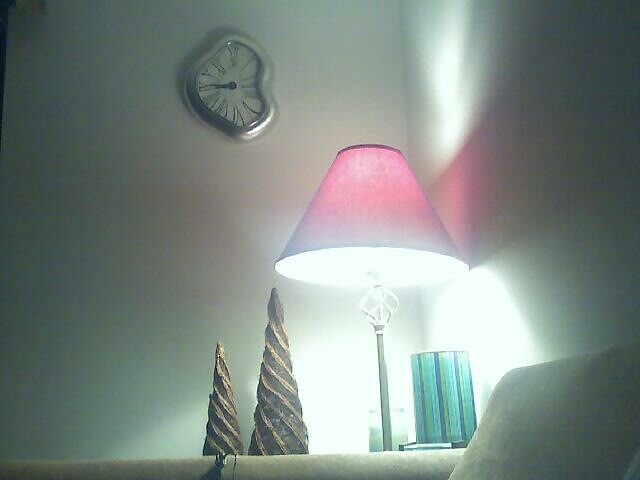In the center of this landscape-oriented image, a stark white wall forms a corner, serving as a minimalist backdrop. Mounted on the wall is an eye-catching, racetrack-outlined clock in lustrous silver. The clock face, distinguished by its Roman numerals, is artistically distorted to mimic the shape of a race track. Dominating the foreground is a pink lampshade emitting a bright white light, anchored by a steel beam that extends downward to the bottom of the frame. The lamp stands adjacent to an intriguing oval-shaped decoration piece, showcasing an abstract blend of green and blue hues. To the left of the lamp, two decorative items resembling grass and miniature Christmas trees add a touch of nature-inspired charm. The bottom edge of the image features the partial view of a green-grey sofa, hinting at a cozy sitting area just out of full view.